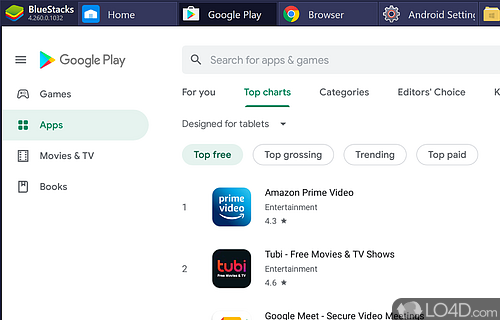This image depicts a user interface of BlueStacks, a software that allows users to run Android applications on a PC. The image specifically showcases the BlueStacks window with several tabs visible at the top: Home, Google Play, Browser, and Android Settings. The user is currently on the Google Play tab, which is highlighted and displays the app's Top Charts.

Within the Top Charts section, the 'Top Free Apps' category is selected. Prominently featured at the top of the list are "Amazon Prime Video" and "Tubi - Free Movies & TV Shows." The third app, "Google Meet - Secure Video Meetings," is partially visible, with the lower part cut off at the bottom of the screen.

In the bottom right corner, there is a watermark reading "load L04D.com," indicating the source where this image may have been originally hosted or captured.

Overall, the illustration provides a snapshot of the BlueStacks interface displaying popular free apps on the Google Play Store at the time the screenshot was taken.